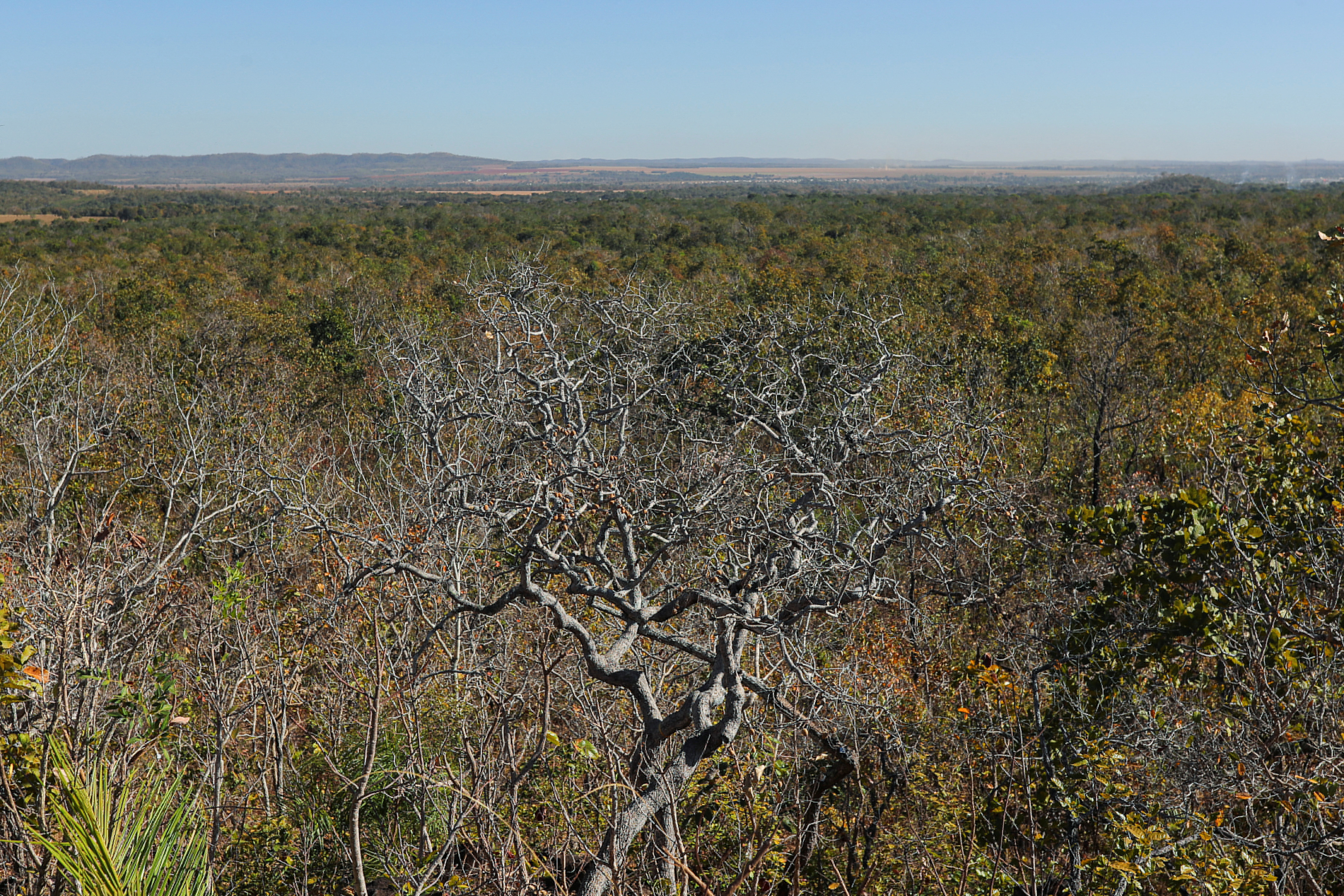The image captures a dry, arid forested landscape taken slightly from above the tree line. In the center of the scene is a thin, wild-branching tree that stands out due to its lack of leaves, contrasting starkly with the surrounding trees which are clad in a mix of orange and green foliage. The forest consists largely of short, shrub-like trees, contributing to an overall dry appearance. To the left, long grassy plants add to the diverse texture. In the background, a line of modest hillside mountains stretches across the horizon, with a few brown, dead grassy fields scattered below, suggesting a parched environment. The sky above is clear and blue, with a hint of haze, yet devoid of any clouds, enhancing the sense of dryness in the scene.